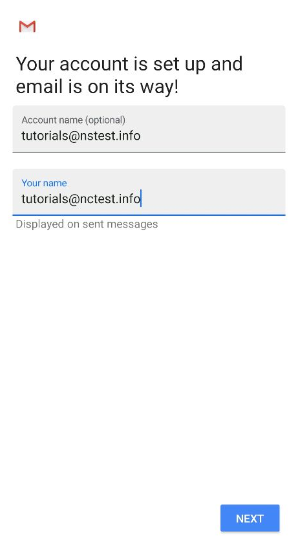The image depicts a clean and minimalist interface for setting up an email account, shown in portrait mode against an all-white background.

In the upper left corner, a prominent email icon featuring a white envelope over a red background is displayed. Directly below it, in large, bold black text, the message reads, "Your account is set up and email is on its way."

Beneath the text, a gray form area is visible. The first field is labeled "Account name (optional)" and is filled with the text "tutorials@nstest.info." Immediately below, the blue-labeled field "Your name" also contains the text "tutorials@nstest.info," with a blue cursor indicating recent activity in this input area, as it is underlined in blue.

Following this form section, there is a subtle, hard-to-read instructional text in gray, "You can be displayed on sent messages," set against the white background, making it less legible.

Finally, after considerable white space at the bottom right corner, there is a conspicuous blue button with "Next" written on it in white text.

The overall context indicates that this is a newly created business email account for nstest.info, with "tutorials" being the user's display name.